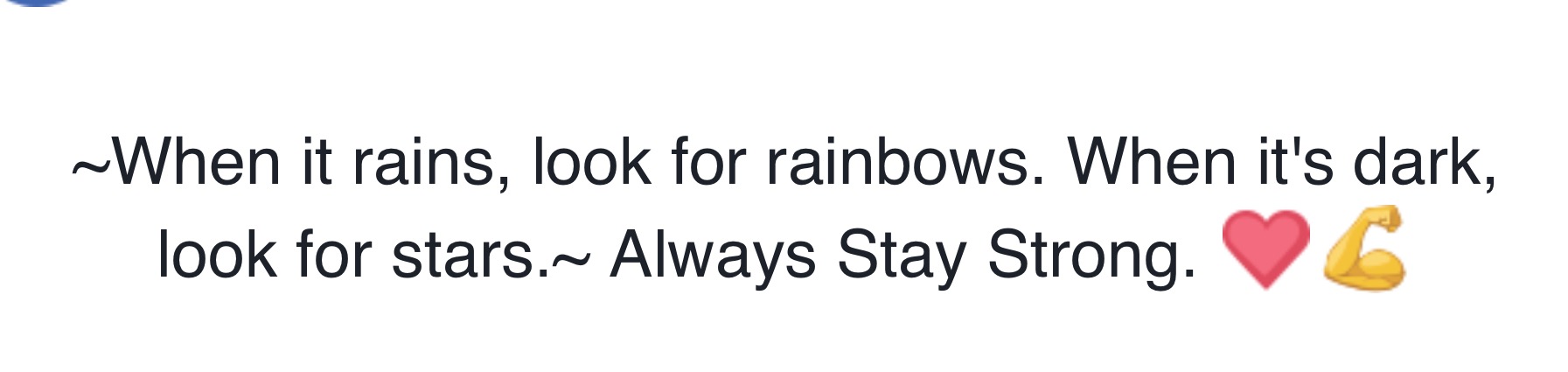The image features an inspirational quote formatted in plain black text on a stark white background. The text begins and ends with a tilde symbol (~), and reads: "When it rains, look for rainbows. When it's dark, look for stars. Always stay strong." Each of the words "Always Stay Strong" is notably capitalized. Accompanying the text are two emojis: a pink heart with a darker pink border, and a flexing bicep emoji. In the top left corner of the image, there is a partial, cut-off circle in purple or blue. The overall appearance resembles a meme or a typical Facebook status update designed to motivate and uplift.